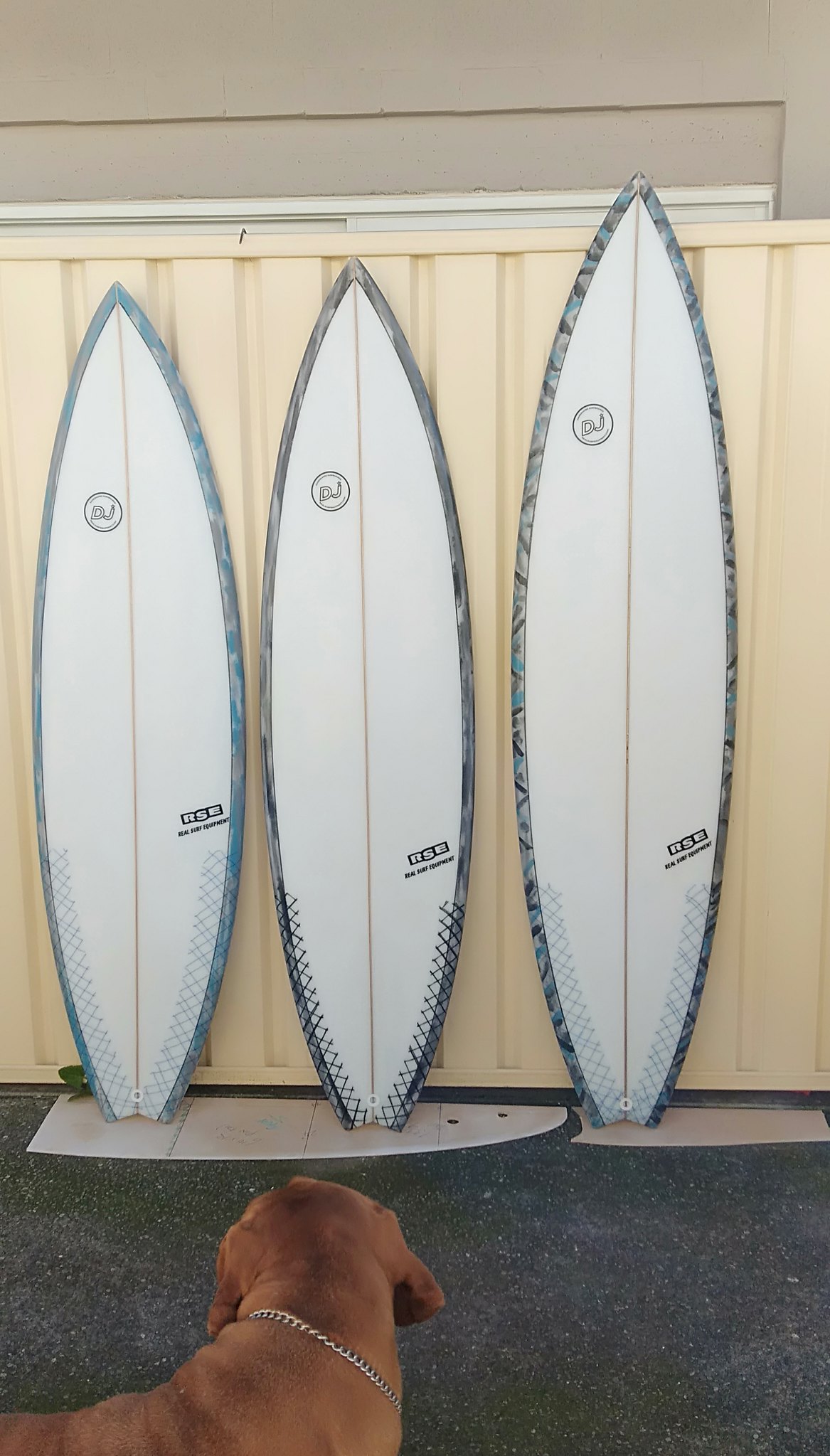In the photograph, there are three surfboards leaning vertically against a light brown or beige wall that appears to be composed of corrugated panels. The surfboards, arranged by height from left (smallest) to right (largest), are predominantly white with distinctive designs. Each surfboard features a light blue border and an orange line running from end to end. The boards also display two stickers, with one near the top that reads "DJ" and another towards the bottom that says "RSE." The ground beneath is covered with dark, spackled tiles reminiscent of a garage or cement floor. In the foreground to the left, a brown dog with a silver chain collar, characterized by droopy ears, gazes intently at the surfboards, positioning itself with its back towards the camera.